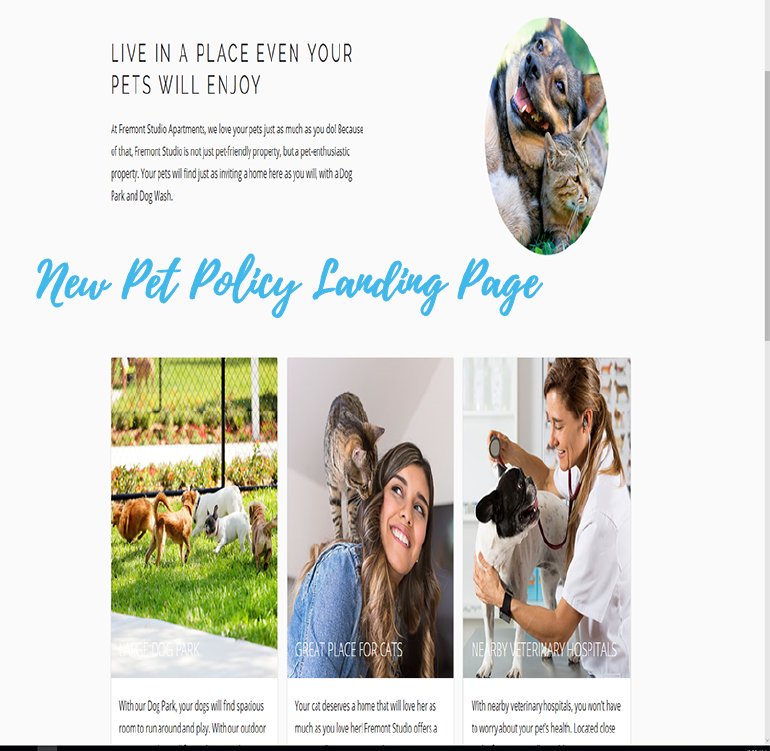The image is from the top left-hand corner of a webpage dedicated to promoting pet-friendly living at Fremont Studio Apartments. The prominent slogan reads, "Live in a place even your pets will enjoy," highlighting the community's dedication to making a welcoming environment for both residents and their furry companions. The caption states: "At Fremont Studio Apartments, we love your pets just as much as you do. Because of that, Fremont Studio is not just pet-friendly property but a pet-enthusiastic property."

In the foreground, a joyful dog is lying on the grass next to a relaxed cat, the dog seemingly smiling with contentment. This image captures the serene and inviting atmosphere that pets can expect at Fremont Studio Apartments. To the right, the text in blue font announces the "New Pet Policy Landing Page," featuring images of multiple dogs running freely in a park.

Additional captions explain the amenities for pets, including a dog park, a dog wash, and spacious outdoor areas for play, though some sentences are cut off. It reads: "With our dog park, your dogs will find spacious room to run around and play with our outdoor," stopping abruptly. There are mentions of nearby veterinary hospitals to assure pet owners of accessible healthcare for their pets. Another incomplete statement starts with "Fremont Studio offers A," suggesting there are additional benefits not fully detailed in the provided text. Overall, the narrative emphasizes the pet-focused features and nearby amenities that ensure a comfortable and enjoyable living experience for both pets and their owners.